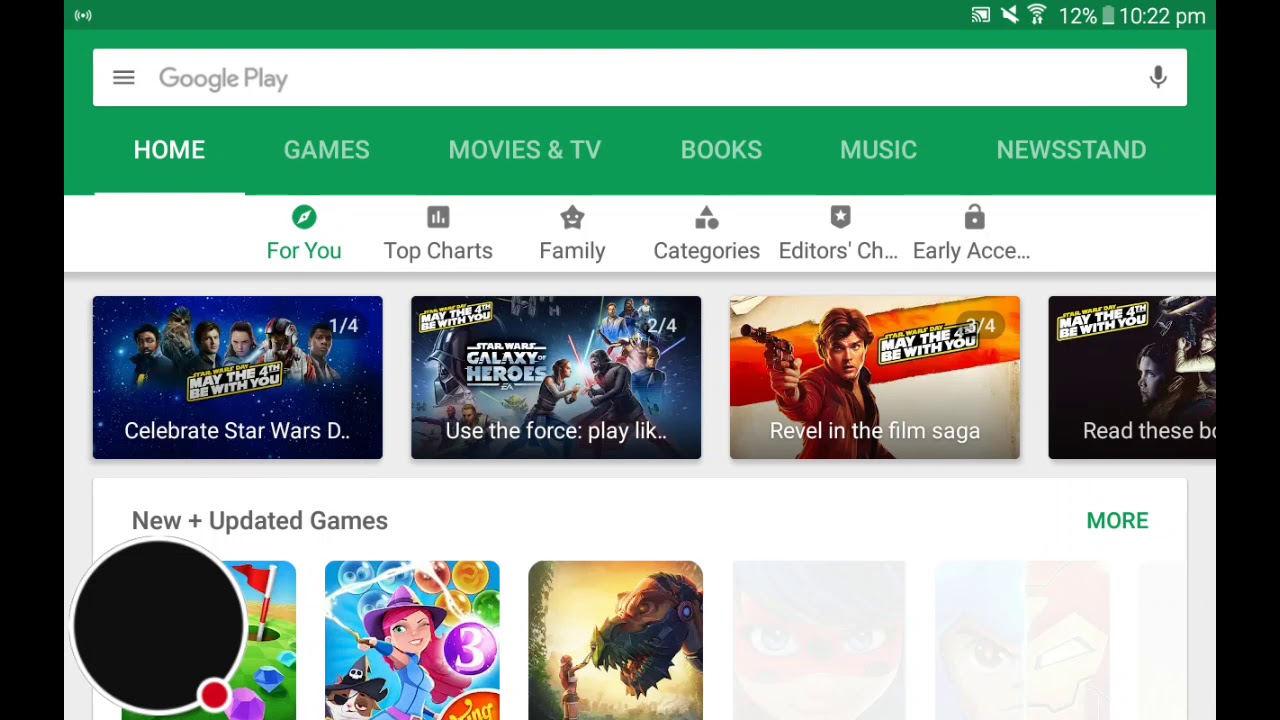The image is a screenshot of the Google Play store interface. The top section features a vibrant green background with the Google Play logo in grey letters. Below this, the main navigation headers are displayed in white text against the green background, including options for Home, Games, Movies & TV, Books, Music, and Newsstand. The Home section is currently selected, indicated by its white highlight. 

The device showing this screen is either a phone or a tablet, as evidenced by the indicators showing a strong connection, muted sound, a nearly depleted battery at 12%, and the time, 10:22 PM.

Beneath the main navigation, additional categories are listed: 'For You' is highlighted in green, while 'Top Charts', 'Family', 'Categories', 'Editor's Choice', and 'Early Access' are in grey text. The last two categories have three-dot menus indicating more options.

Promotional content below these categories features a blue banner with "May the 4th Be With You" to celebrate Star Wars, including phrases like "Celebrate Star Wars," "Our Wars," "Galaxy Heroes," and "Use the Force." The promotion repeats the tagline "May the 4th Be With You," with varying calls to action such as "Revel in the Film Saga" and "Read the Something," indicating a cut-off text.

Further down, the "New and Updated Games" section showcases various game thumbnails: one with a golf course adorned with jewels, another featuring a witch or sorceress casting bubbles, a cat in a pirate hat, and a woman reaching out to a dinosaur restrained by a muzzle. This comprehensive view highlights the available games and the overall layout of options within Google Play.